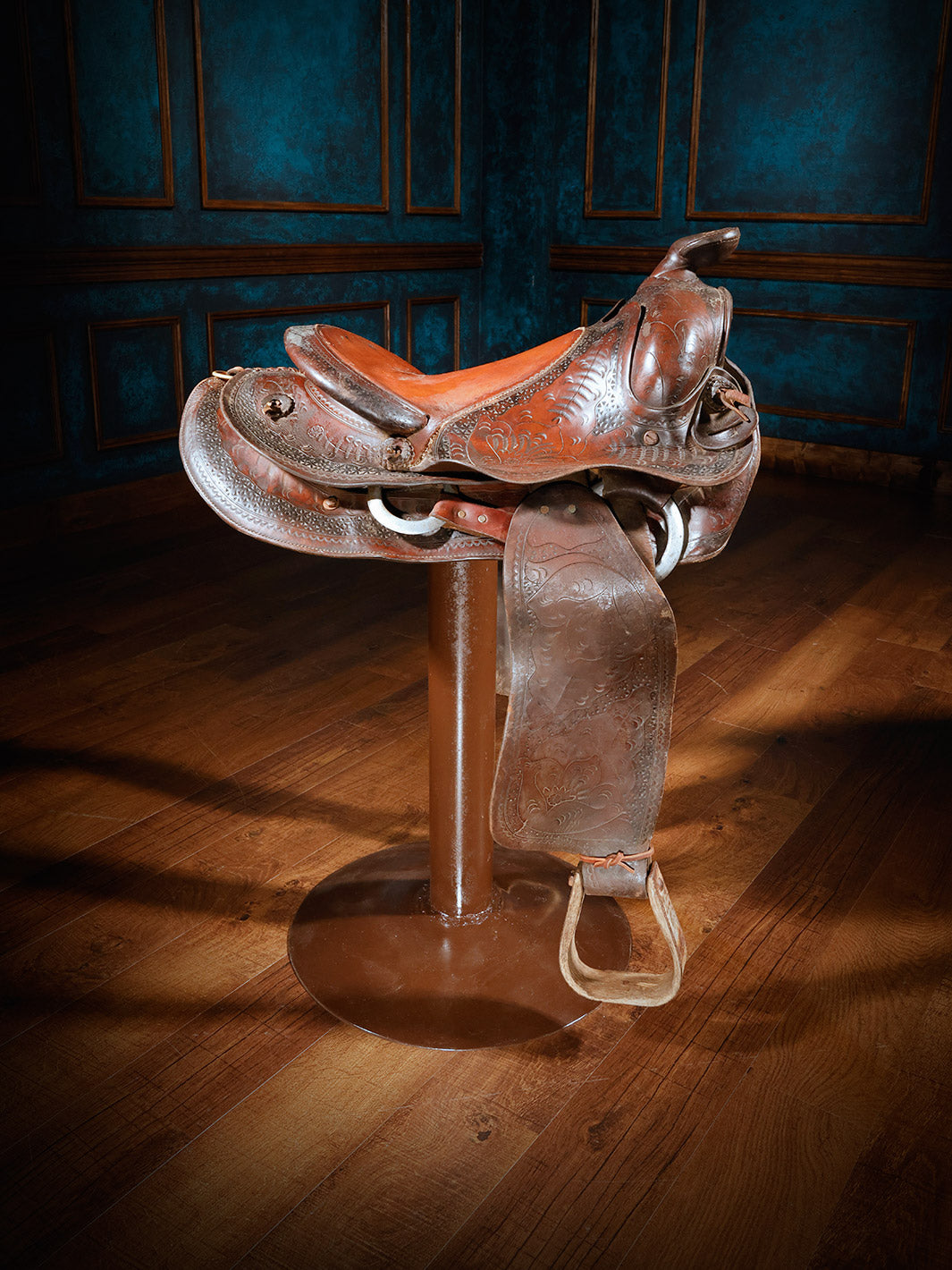The image features a well-worn, leather horse saddle illuminated by a focused light that highlights its details, making the textures and colors stand out. The saddle, predominantly a reddish dark brown except for its lighter, more reddish tan seat, is positioned on a brown metal stand. The saddle's horn is situated to the right of the image, while the stirrup faces the viewer directly in an open and accessible manner. The scene takes place on a plank wood floor and is set against a darker blue wall with medium dark stained wood trim, adding a warm and rustic atmosphere to the room.